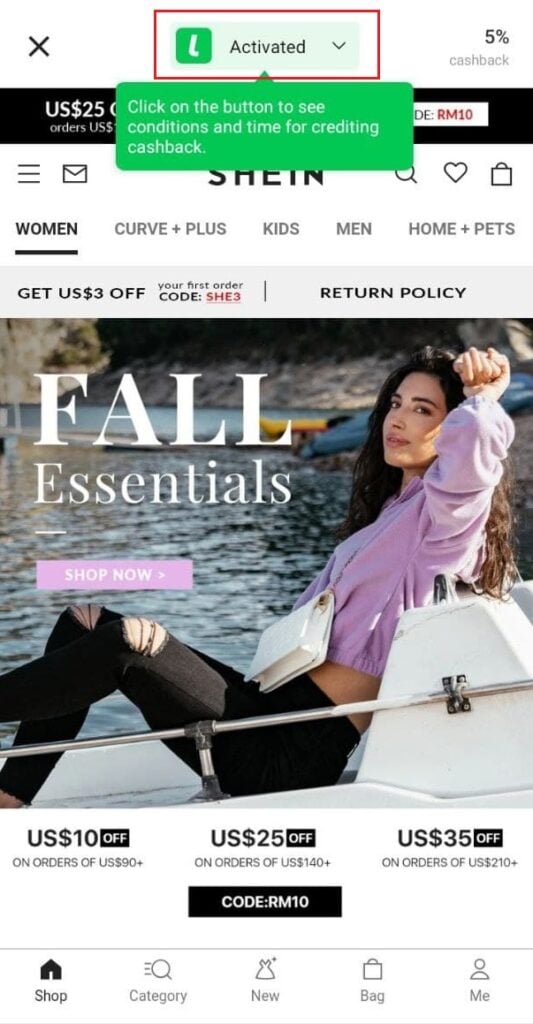In this image, there is a screenshot of the SheIn app displayed on a smartphone. At the top of the screen, there's an "X" button, presumably for closing the app or the current screen. Below the "X," the word "Activated" is prominently displayed with a drop-down arrow next to it, in black font. 

Centrally located, there is an icon composed of a white "L" on a green square, with a red outline around the square. Below this icon, a green bubble notification with white text states: "Click on the bottom to see conditions and time for crediting cashback."

To the right, "5% Cashback" is visible, although some of the text at the top is partially obscured by the green notification bubble.

Scrolling further down, the app's navigation menu is open to the women's section, with additional categories visible, including "Women," "Curve + Plus," "Kids," "Men," and "Home + Pets." 

A promotional banner offers "$3 off when you use a certain code," and features an image of a woman sitting on a boat, accompanied by the text "4 essentials."